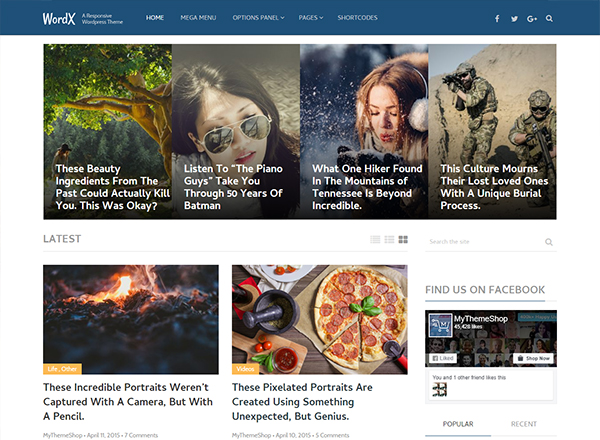**Detailed Caption:**

The image showcases a webpage from WordX, a progressive WordPress theme. The page's header features a navy blue text box at the top bearing the WordX logo, followed by an unreadable tagline due to blurriness. The navigation menu includes options titled Home, Mega Menu, Options Panel, Pages, and Shortcodes, with Options Panel and Pages being dropdown menus. To the right of these options, there are icons for Facebook, Twitter, Google+, and a search magnifying glass.

Beneath the navigation bar, the screen displays a row of four images labeled "Latest." The first image depicts a tree and carries the caption: "These beauty ingredients from the past could actually kill you. Was this okay?" The second image shows an Asian woman wearing sunglasses and looking upwards, accompanied by the text: "Listen to the piano guys take you through 50 years of Batman." The third image features a woman with earmuffs blowing ice off a glove, and the caption reads: "What one hiker found in the mountains of Tennessee is beyond incredible." The final image in the row displays two soldiers shooting in a desert setting, with the caption: "This culture mourns their lost loved ones with a unique burial process."

Below these images, there are additional visuals including one of what appears to be fire on burning coals, another of a pizza, and a "Find us on Facebook" prompt.